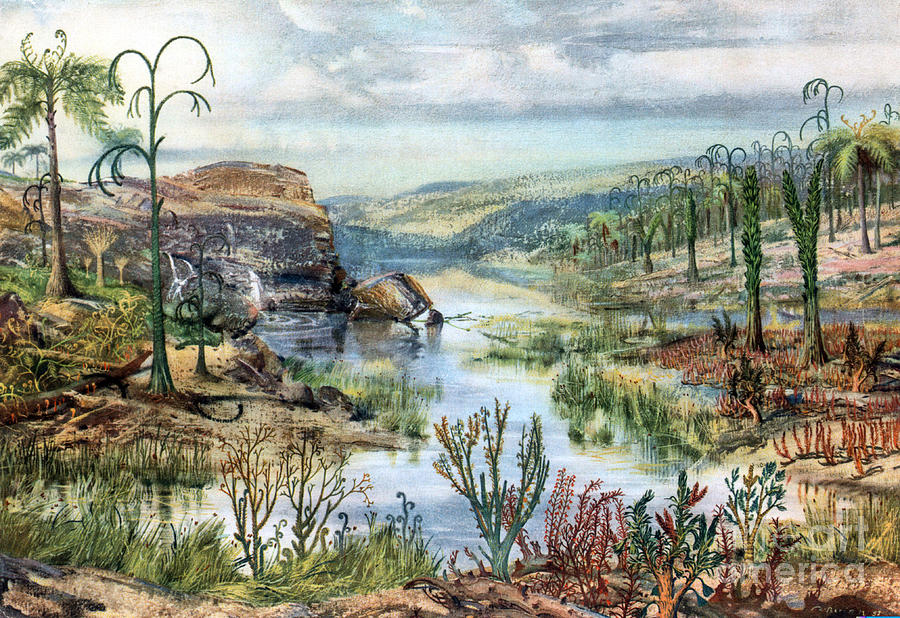This detailed painting, possibly an acrylic or oil piece, portrays a surreal prehistoric landscape, emphasizing the imaginative and non-modern plant life. In the foreground, various desert succulents are depicted, with green, arm-like stems and some maroon-colored plants with tiny dotted limbs. This barren, brown land transitions to a wetland-seeming river or lake at the center, banked by shoreline scrub brush. On the right, fantastical, skinny trees rise up, including leafless ones with circular branches and a prototypical palm tree with just four fronds. Behind this scene are low-lying, greenish-yellow mountains, contrasted by a pale blue sky streaked with white clouds tinged with gray. The unique trees and plant life—ranging from fern-like green plants to long grasses—are unlike any seen today, adding to the prehistoric or fantasy ambiance of the scene.